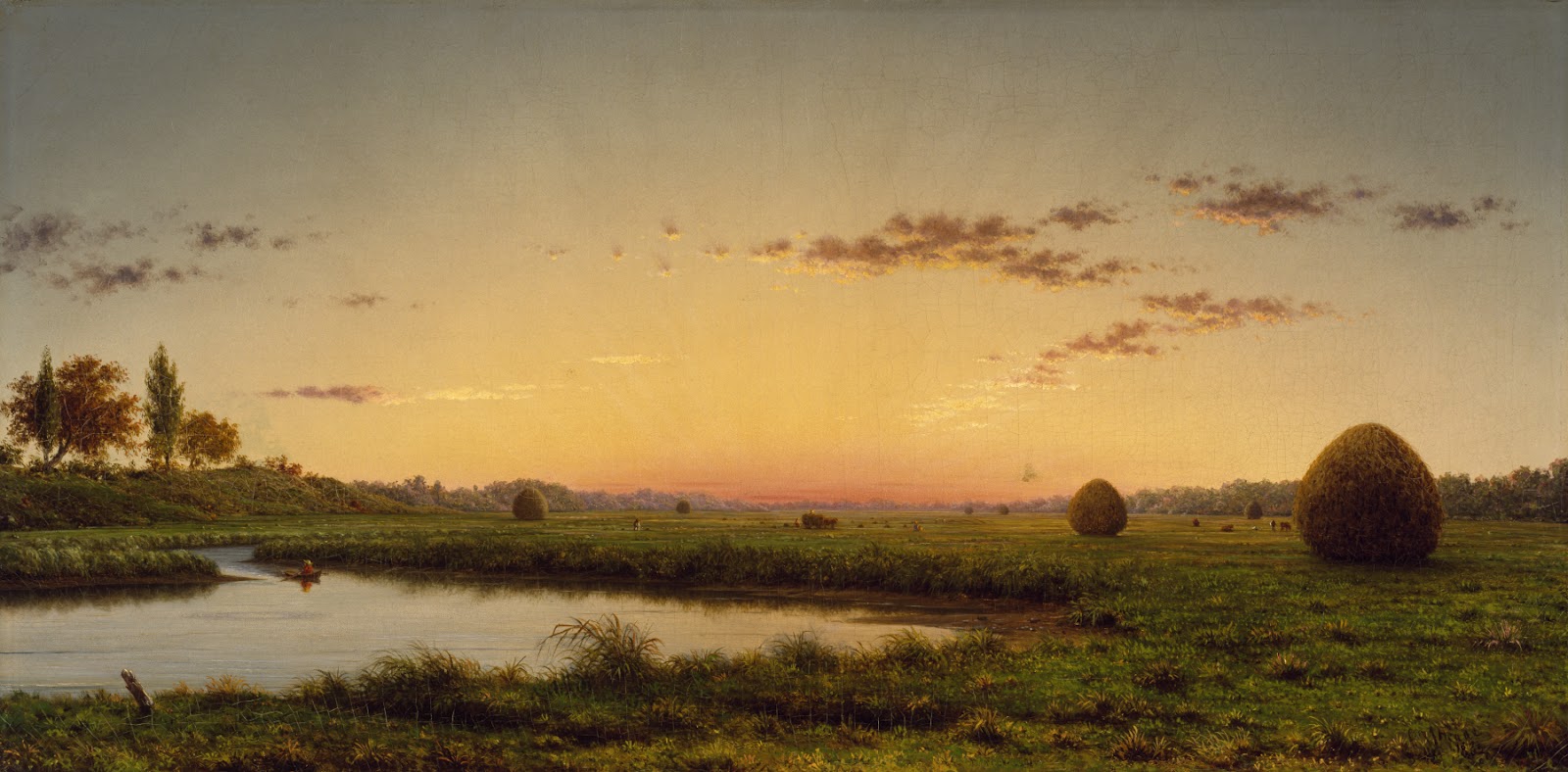The image captures a serene natural landscape at sunset, characterized by a richly detailed painting. On the left side of the image, there is a gentle mountain slope topped with two tall green trees and two wider brown trees. Below this slope, a small, meandering river flows from the left towards the center of the image, bordered by lush, grassy banks. Midway through the image lies a tiny pond. The background of the landscape reveals a series of dome-shaped, brown structures that resemble grass huts or bales of hay, dotting the expansive field which stretches far into the distance. On the right side, there are more hills adorned with trees, vegetation, and wildflowers. The sky, occupying about 75% of the image, boasts a stunning display of a colorful sunset in hues of pink, red, and yellow with a few scattered clouds, enhancing the natural beauty and tranquility of the scene.